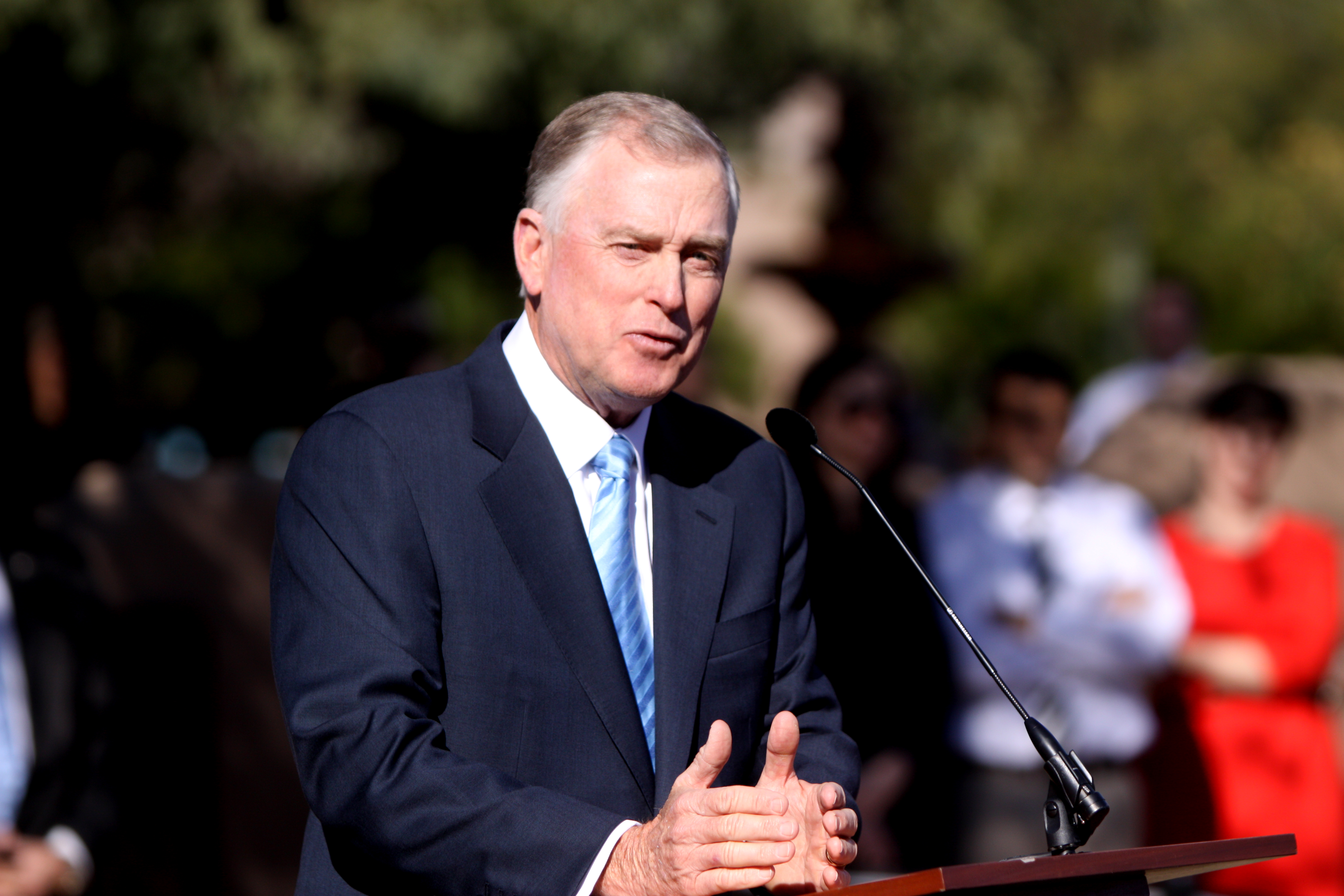A white male in his 50s, with gray hair and a fair complexion, stands at a wooden podium outdoors, in what appears to be midday sunlight. He wears a navy blue business coat over a white, button-collared shirt, and a light blue tie with white stripes. His hands are positioned on the podium, almost as if holding an invisible cup, with his thumbs up, suggesting a gesturing motion. His mouth is slightly open, forming a semi-smile, indicating he is speaking. His eyes are squinted, likely due to the sun shining in his face. Behind him, the background is blurred, showcasing green trees and several people, some with arms crossed, dressed in various colors including red, white, and dark shades, all appearing to focus on him. A thin black microphone is affixed to the podium, angled towards his mouth, capturing his speech. His shoulders are slightly angled, and he looks towards the right of the camera, not directly into it.